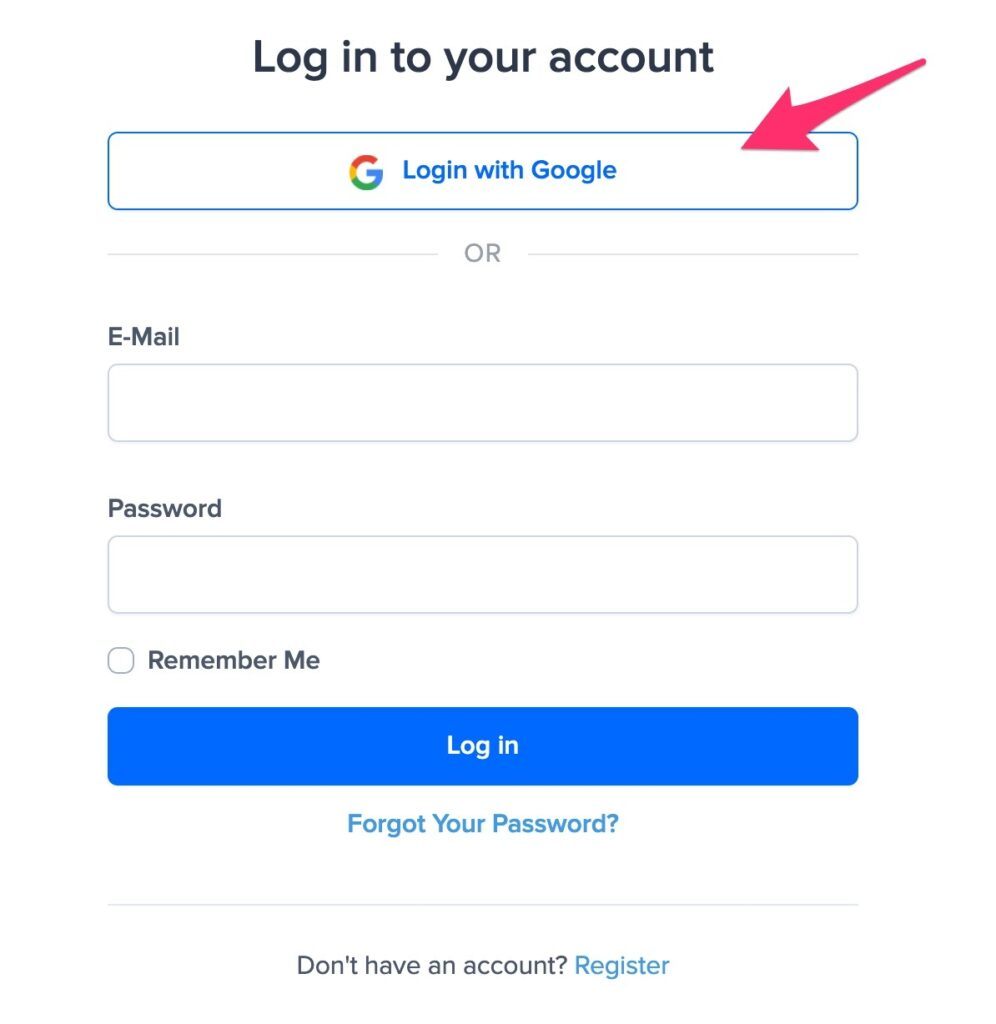This image depicts a Google login page. At the top, in bold black text, it prompts users to "Log into your account." Below this text is a prominent blue rectangle featuring the Google logo and the text "Log in with Google," highlighted by a pink arrow pointing towards it. 

Following this, in subtle gray text, the word "or" separates the Google login option from the traditional email login fields. Underneath this, there is a series of two gray rectangular boxes; the first is labeled "Email" and the second "Password." Beneath the password box, a small checkbox labeled "Remember me" is situated.

At the bottom of the form, a larger blue rectangular button with the same dimensions as the previous boxes displays the text "Log in." Below this button, the phrase "Forgot your password?" appears in turquoise text. A dividing line separates this section from the final prompt, which reads "Don't have an account? Register."